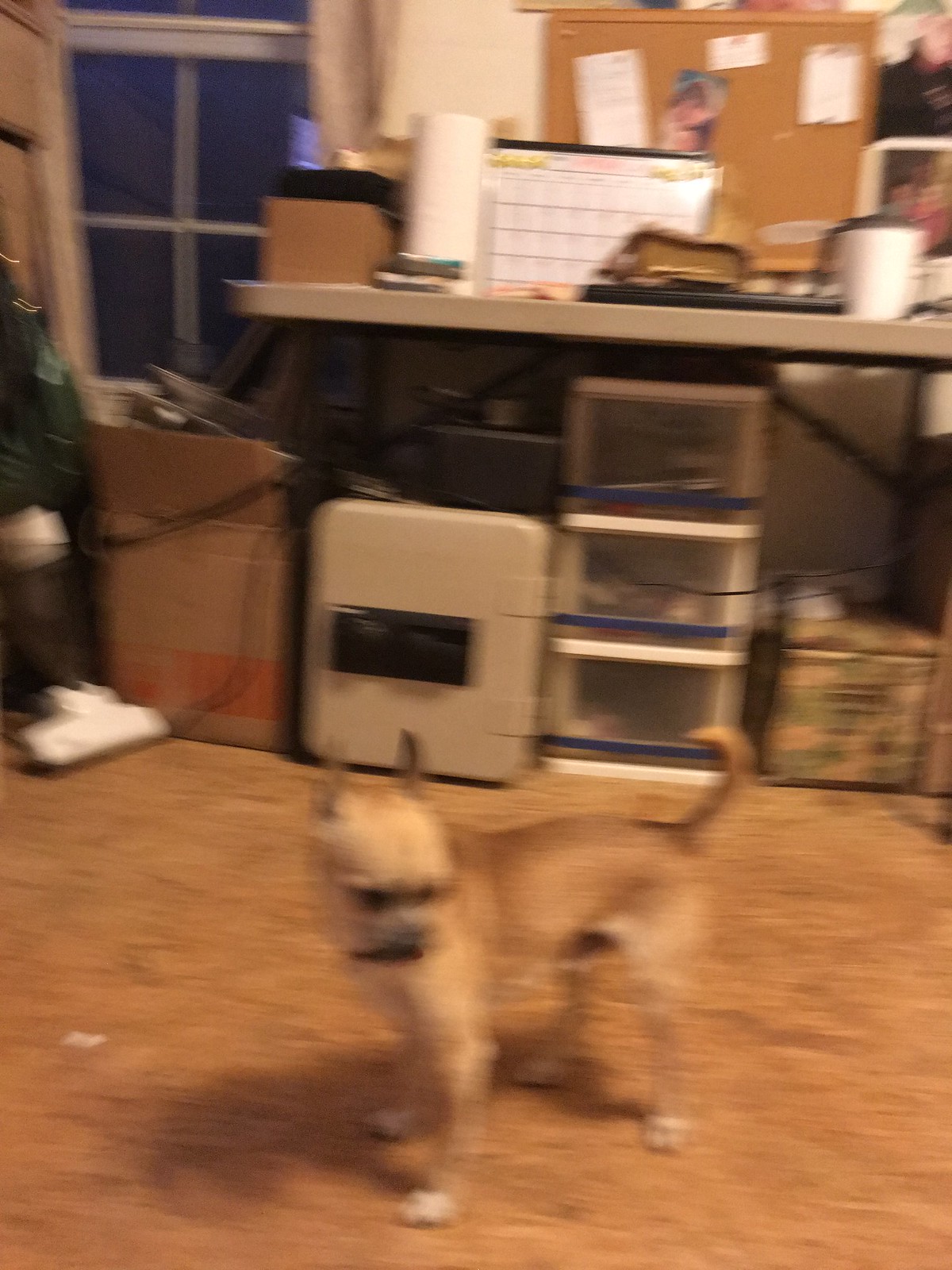In this blurred photograph, we are presented with a vertically oriented image capturing the interior of a worn-out room or possibly an office. The surroundings appear shabby and cluttered, creating an uneasy atmosphere. On the right side of the image, a beige shelf or desk-like unit is barely detectable amidst the blur. Atop this unit lies a paper towel roll and a paper calendar. The backdrop features a corkboard adorned with various irregularly shaped papers pinned haphazardly.

The focus of the image, however, rests on the lower center where a small dog, possibly a puppy, is visible. The dog has a tan coat and is depicted in a side profile stance, with its head turned to the right and its body facing left. Beneath the desk area, there is a small, shabby-looking refrigerator with visible dirt on its surface, accompanied by a three-drawer plastic shelving unit that adds to the room's disheveled appearance.